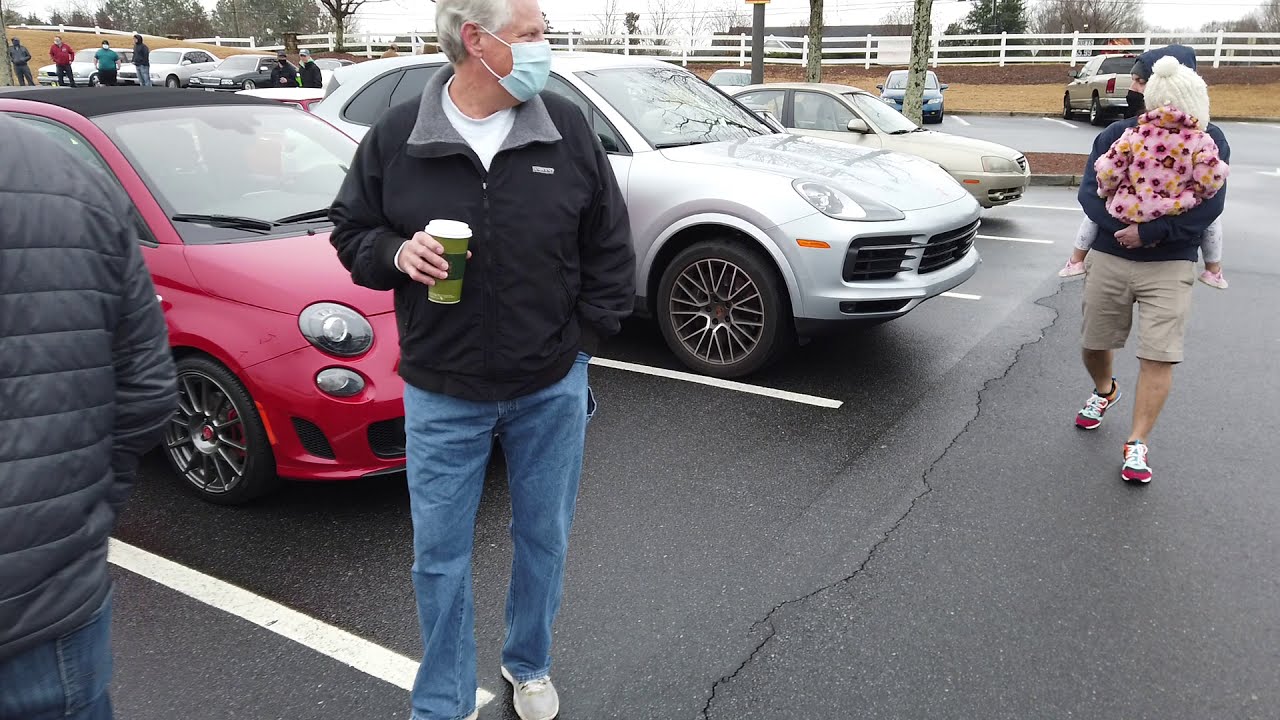In the detailed photograph of a parking area, three individuals can be seen. To the left, a man with his back to the camera wears a black coat and blue jeans, visible by his shoulder and pants. In the center, an older gentleman, with gray hair and a blue surgical mask, stands holding a green cup of coffee in his right hand. He's dressed in a black jacket, white t-shirt, and blue jeans, with gray tennis shoes. On the right, another man, carrying a small child in his arms, walks towards the center man. This man is cloaked in a blue hoodie, beige shorts, and maroon shoes, with a black mask partially obscuring his face. The child he carries is outfitted in a pink coat adorned with floral patterns and a white hat with a pom-pom. Surrounding them, three cars are parked prominently: a red car, a silver SUV, and a beige sedan. In the distant upper left corner, another row of cars can be seen, with people mingling in front of them. The parking lot itself is asphalt, showing a noticeable crack running through the center toward the right, and white lines marking the parking spaces. A white fence with wooden planks extends across the background.